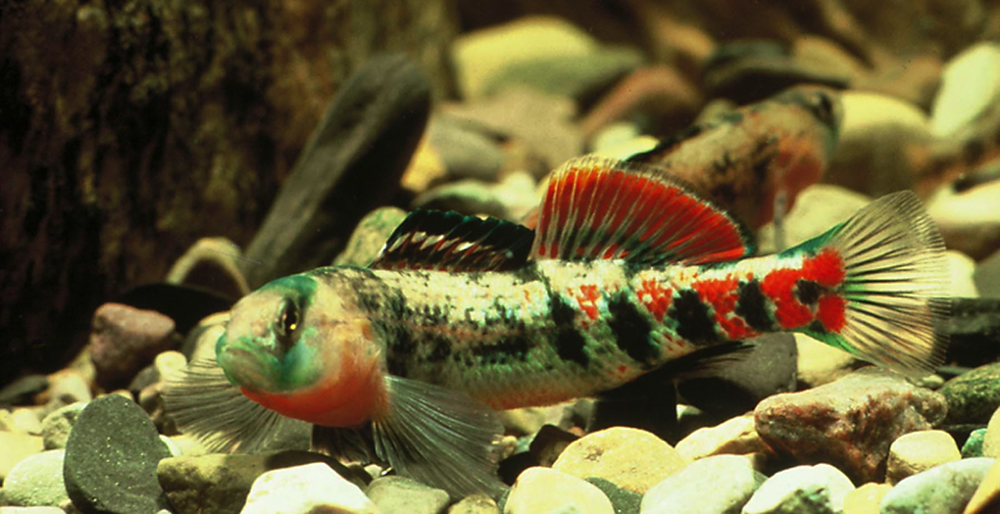The close-up photo captures a single small fish swimming above a varied collection of small rocks. The fish's long, scaly body is a predominantly light gray, punctuated by vivid patches of black, red, and turquoise stripes and blotches. Its head faces the viewer, showcasing a white face and mouth with hints of orange beneath. The fish has two front fins that appear translucent with tinges of gold, and its dorsal fins feature a combination of black, white, and orange. Another fin at the back is similarly colorful, and the fish's overall body displays a shimmering silvery gold hue with green and red patterns. In the background, the scene includes smaller and larger rocks of gray, white, tan, and reddish-brown colors, and a dark brown tree-like structure with a bark-like texture, adding a naturalistic depth. The water is so clear that it seems almost invisible, creating an impression of murkiness further back where muted green tones suggest underwater plants or coral.